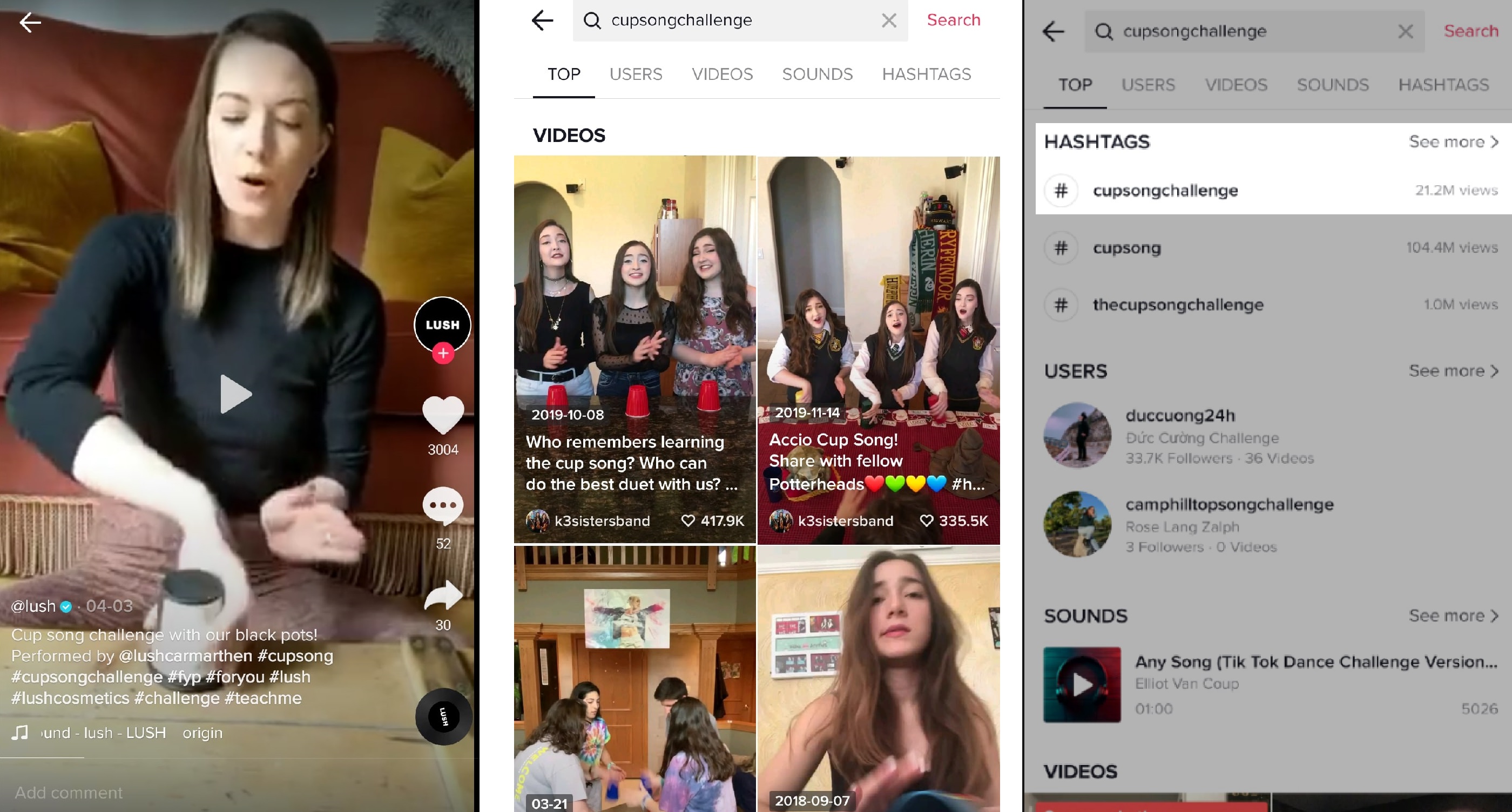In the image, a woman is seen with her hand turned, holding an upside-down cup. This appears to be part of a video interactive experience with a "cup song" theme, as hinted by the hashtag #CupSong. When clicked, the arrow promises the viewer the full video, revealing what she intends to do. The caption indicates that the middle video invites viewers to learn the cup song and participate in duets, asking, "Who recommends learning the cup song? Who can do the best duet with us?"

Additionally, the image features thumbnails of other cup song-related videos:
1. The first video shows a woman at home performing the cup song behind a couch with pillows, using a coffee table.
2. The next video features three girls, possibly in school uniforms, performing the cup song in a home-like setting, and encourages viewers to share and follow. Notably, it has four heart icons in red, green, yellow, and blue.
3. Another clip shows women at a table engaging in an activity with cups, though it lacks a descriptive label.
4. The final video presents a girl with long brown hair, who is presumably performing the cup song, though the content is not explicitly labeled as such.

The collective depiction of these scenes emphasizes a communal and interactive experience centered around the popular "cup song" activity.